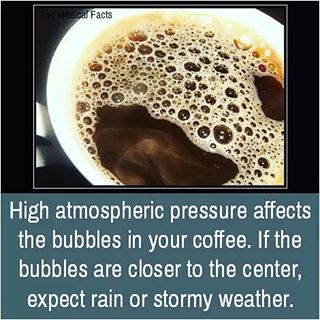The image resembles a meme and consists of two distinct parts. The top half showcases a close-up photograph of a white coffee cup filled with brown coffee, displaying noticeable bubbles or foam clustered toward the center of the cup. The background behind the coffee is black, with a tiny, hardly discernible text at the very top, featuring the word "FACTS" just visible above the coffee cup. The side of the cup appears slightly stained a light beige. The bottom half of the image features a bluish-gray/teal background with a block of white sans-serif text that reads: "High atmospheric pressure affects the bubbles in your coffee. If the bubbles are closer to the center, expect rain or stormy weather." The white text spans the entire bottom portion, reminiscent of a meme's design, coupling the informational content with the visual emphasis on the coffee bubbles.